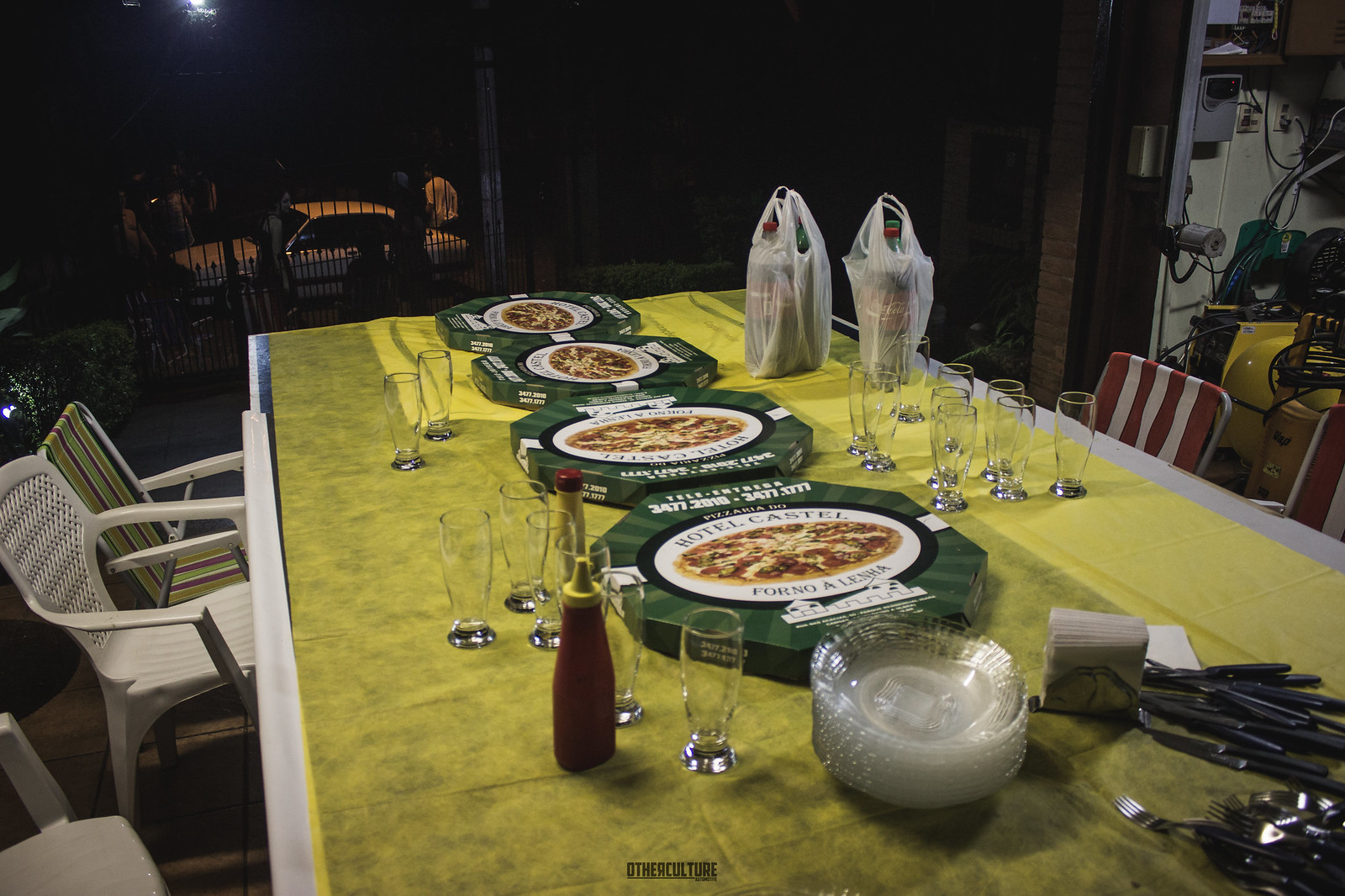This color photograph depicts a long dining table that is angled from the bottom right to the top left. The table is predominantly white with a yellow runner extending the length of the table, which is adorned with various items suggesting a casual gathering. Central to the arrangement are four closed, green pizza boxes arranged diagonally, each shaped somewhat like stop signs. Each box features a white circle with a pizza image and some indistinguishable text, likely the store name and type of pizza.

The scene is somewhat washed out and may have a green and yellow tinge, possibly due to a filter. Around the table, there's an eclectic mix of mismatched outdoor chairs, including white plastic ones and others with webbing and red-and-white stripes. Various items are scattered across the table, including glass goblets for beer, a bottle of either sriracha or ketchup on the left, and two white plastic bags in the center with liquor bottles peeking out. A glass bowl containing a white creamy substance is positioned near the lower right corner, with piles of plastic plates and cutlery nearby.

The background is dark and not well-lit, revealing the presence of a brown area through a wrought iron gate, leading to a street with a white car parked. There are also indications of possible electrical settings and some other indistinct yellow objects in the far right corner, adding to the overall casual yet somewhat cluttered appearance of the scene.